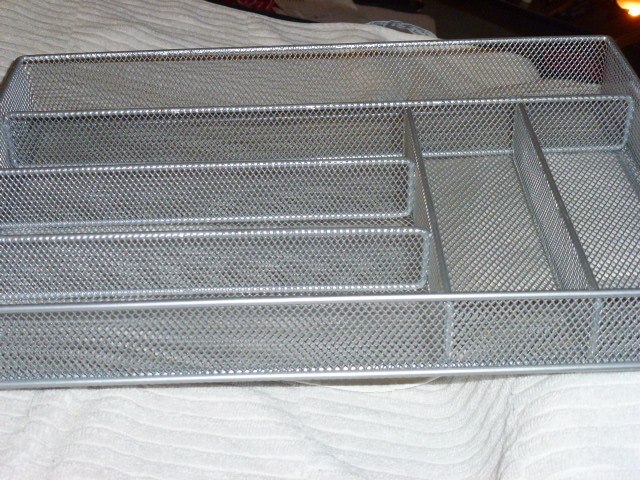This photograph showcases a rectangular drawer organizer constructed from a brushed silver or nickel wire mesh in a fence-like design. It features six compartments: four horizontal sections, one of which spans the entire length of the organizer, while the other three occupy about two-thirds of the length. These are intersected by two vertical compartments, creating a versatile arrangement for organizing items such as silverware, pens, or pencils. The organizer is placed on a white, textured fabric surface, perhaps a blanket or a towel, and the photo appears to have been taken indoors with the aid of a flash, illuminating the empty container.